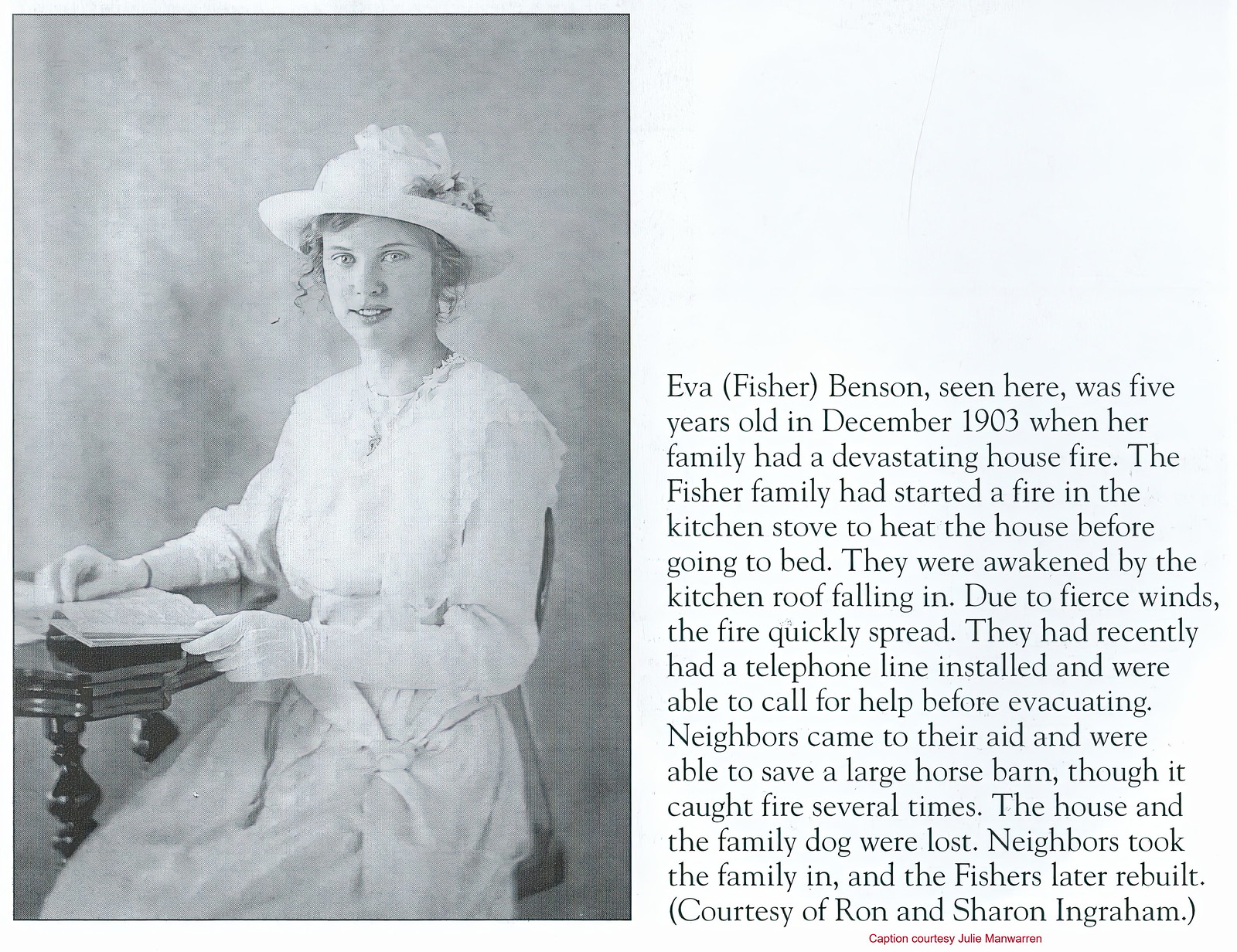The image features a young woman seated on the left side of the frame. She is gracefully dressed in a white dress, white gloves, and a bonnet, with tendrils of her hair cascading out from under the hat. Her body is turned toward the left edge of the image, and she is seated at a table with an open book. She is looking directly at the camera, her left hand resting on the open book and her right hand placed on it as well. Around her waist, there is a sash, adding an elegant touch to her attire. On the right side of the image, there is a detailed paragraph of text that provides information about her. The text introduces her as Eva Fisher Benson, who was five years old in December 1903 when her family experienced a devastating house fire. The Fisher family had lit a fire in the kitchen stove to heat their home before going to bed, only to be awakened by the kitchen roof collapsing due to fierce winds. The fire rapidly spread, but they had recently installed a telephone line and were able to call for help before evacuating. Neighbors assisted and managed to save a large horse barn, despite it catching fire multiple times. Tragically, the house and their family dog were lost. Generous neighbors took the Fishers in, and they later rebuilt, thanks to the support of Ron and Sharon Ingraham.